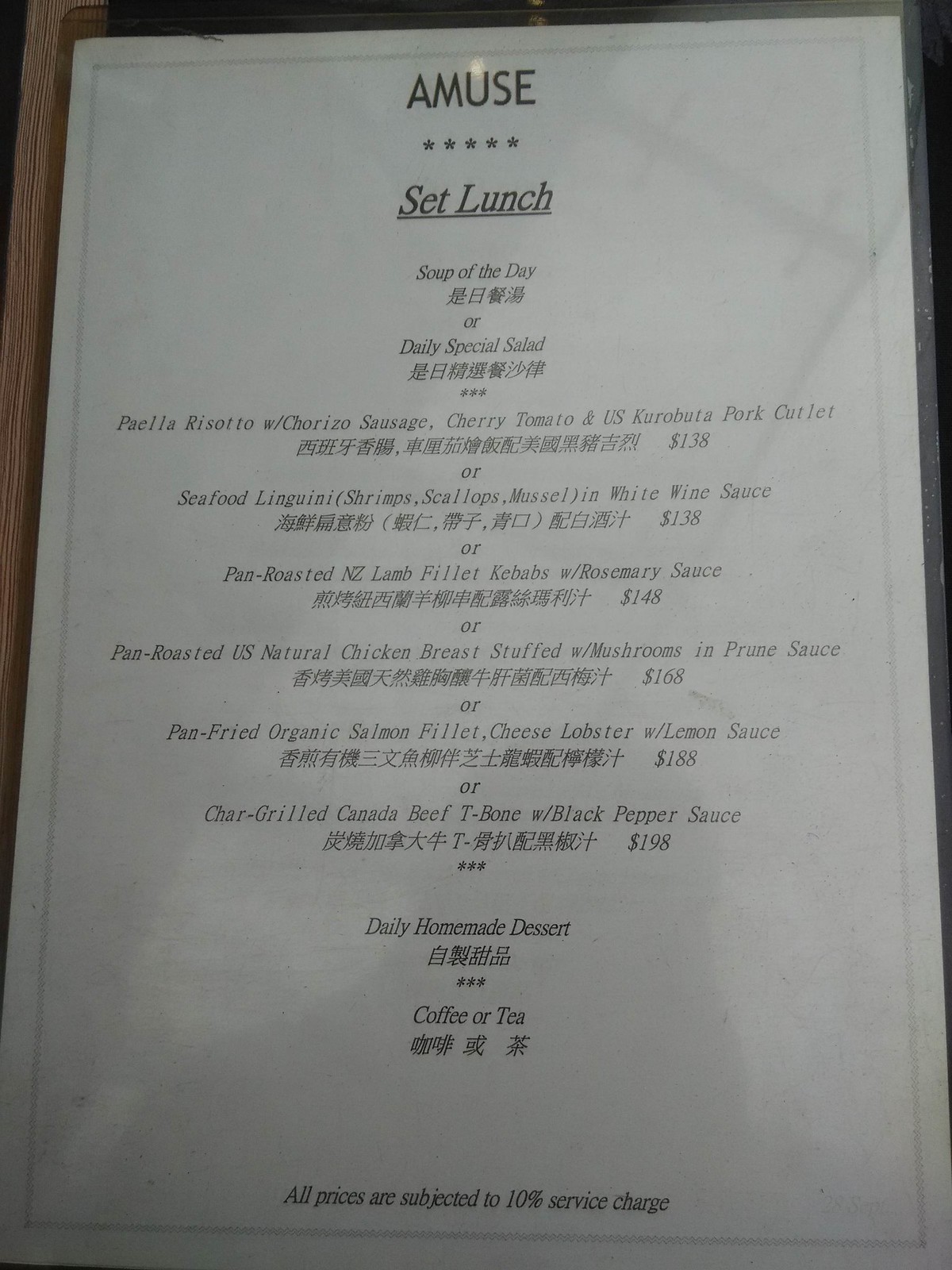The image portrays an indoor scene featuring a restaurant menu placed atop a medium brown-colored table. The menu itself is white with black text and prominently displays the name of the restaurant, "A Muse," which is accompanied by a five-star rating at the top. The menu is titled "Set Lunch" and includes various food offerings, starting with a "Soup of the Day" and a "Daily Special Salad." Below the English descriptions, there are Chinese characters. The menu lists several main courses: "Seafood Linguine with Shrimp, Scallops, Mussels, and White Wine Sauce" priced at $138, "Pan-Roasted NZ Lamb Fillet Kebabs with Rosemary Sauce" at $148, "Pan-Roasted U.S. Natural Chicken Breast Stuffed with Mushrooms and Prune Sauce" for $168, and "Pan-Fried Organic Salmon Fillet with Cheese Lobster and Lemon Sauce" at $188. For dessert, it offers a "Daily Homemade Dessert," along with coffee or tea. A note at the bottom indicates that all prices are subject to a 10% service charge.